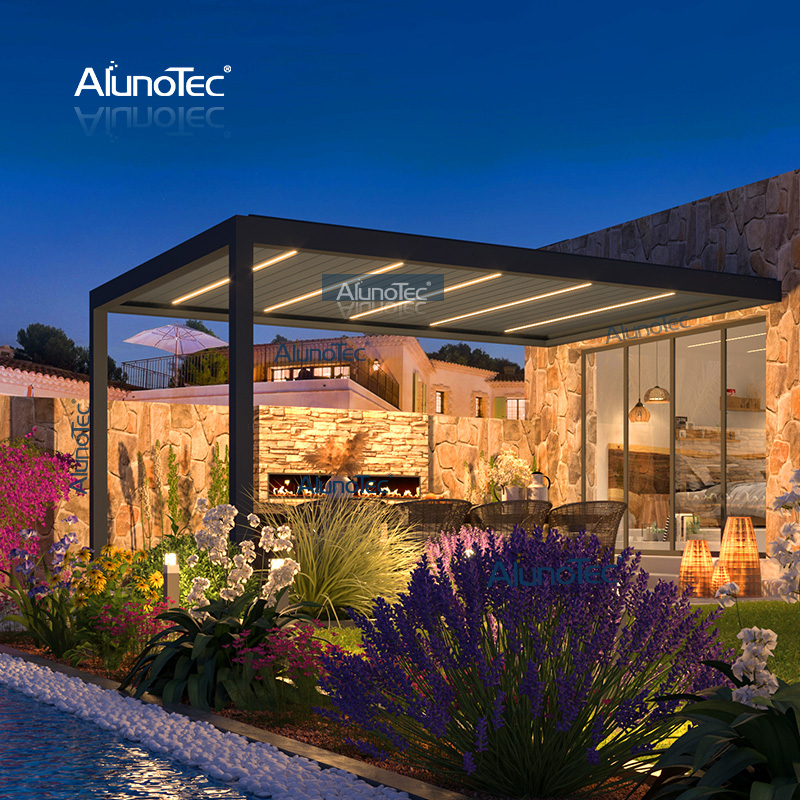This image captures a modern and elegant house at night, beautifully illuminated under a dark blue sky. The top of the picture prominently displays the name "Alunatec" and a mirrored shadow effect below it, possibly indicating a brand associated with the structure or its lighting design. On the right side of the frame stands the stone house featuring extensive glass patio doors, which offer a view inside to a well-lit room that may be a bedroom. The patio extends to the left, covered by an overhang or awning that also bears the name "Alunatec."

Below the awning, there's an outdoor seating area, illuminated by several lights, and a light brick fireplace with an active fire, adding to the cozy ambiance. Surrounding the patio, a carefully maintained garden blooms with a vibrant array of pink, purple, and green flowers, featuring different types of bougainvillea and other decorative plants. Adjacent to the garden, on the left side of the image, there's a hint of water, suggesting the presence of a pool.

Overall, the photograph exudes a sense of high-quality craftsmanship and modern design, showcasing a harmonious blend of natural elements and sophisticated architectural details.